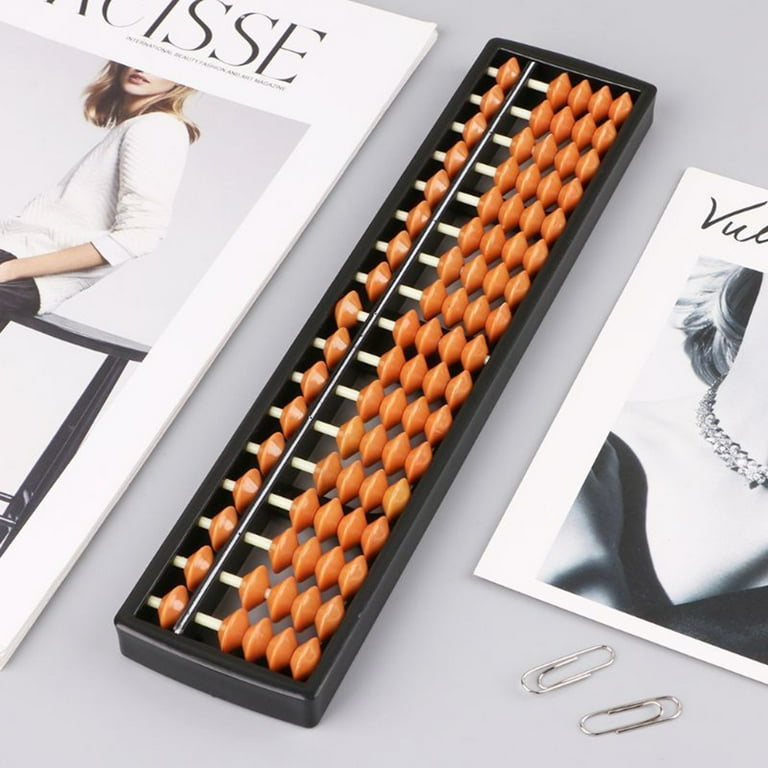The image depicts a modern gray work desk adorned with a variety of items. On the left side of the desk, there is a fashion magazine featuring a woman in a white shirt perched on a black stool, with the last four letters on the cover spelling out "I-S-S-E." Central to the composition is a tall, black rectangular object resembling an abacus, filled with rows of orange wooden beads. To the right, the desk holds two large paperclips positioned under a black and white headshot of a woman, showcasing a necklace. The photograph partially reveals the woman’s neck and light blonde hair, with traces of the cursive letters "V-U-L" visible above. Together, these elements create a meticulously arranged scene on the sleek, gray surface of the desk.